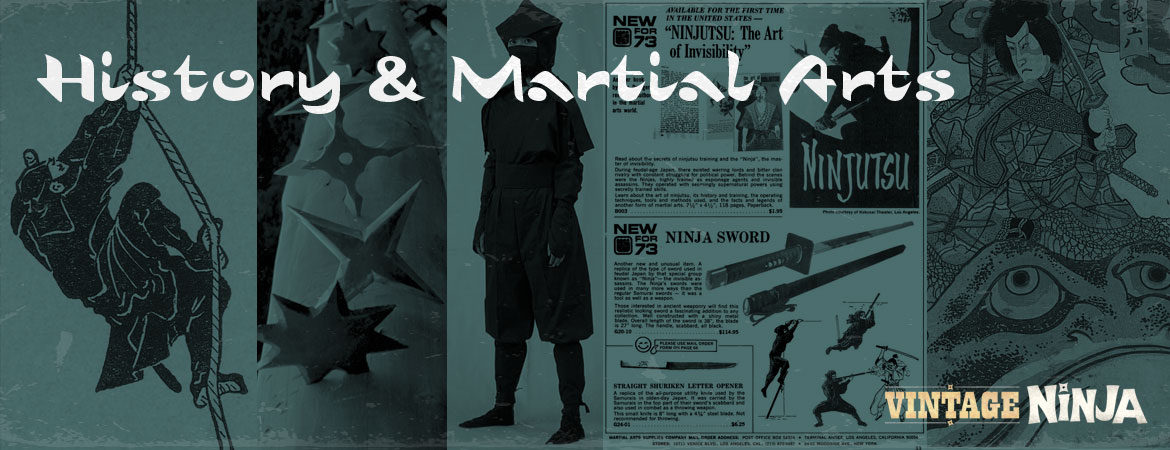The image is a detailed, blue-filtered collage focused on ninja martial arts and history, giving it a vintage feel. At the top left corner, bold white text reads "History and Martial Arts," while in the bottom right corner, "Vintage Ninja" appears in smaller, alternating brown and white text. The background features a dark greenish-blue and grayish-teal color scheme. On the left side, a detailed drawing shows a ninja in black attire, skillfully climbing a rope using flexible shoes. Adjacent to this, a photograph displays a variety of ninja throwing stars, ranging from sunburst designs to circular blades. Further to the right, traditional Japanese-style art complements the composition. Central to the image is an article about ninja swords. The overall structure suggests an infographic or promotional material, possibly from a book or a page dedicated to the history of martial arts.